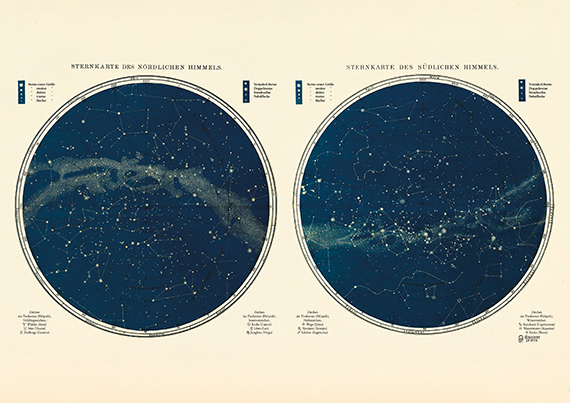This is an image of star charts that appear to be a detailed poster diagram in a Scandinavian language, likely stating "Sternkarte des Nördlichen Himmels." The background of this diagram is white, and it features two large, side-by-side circular sections, reminiscent of views through binoculars or a telescope. Both circles prominently display star charts against a deep blue background with numerous white stars, some of which form constellations connected by thin lines. There are intricate, faint smears indicating the Milky Way: in the left circle, it arches upwards, while in the right, it forms a smile-like curve. The circles are surrounded by text labels and descriptions that are too small to read clearly but likely describe the parts of the night sky depicted. The charts include some additional detailing like asteroid belts or cloud/water covers. The entire diagram is topped with a title in a pink hue. This meticulously rendered star chart captures various aspects of the northern sky, offering different views presumably for different times or seasons.